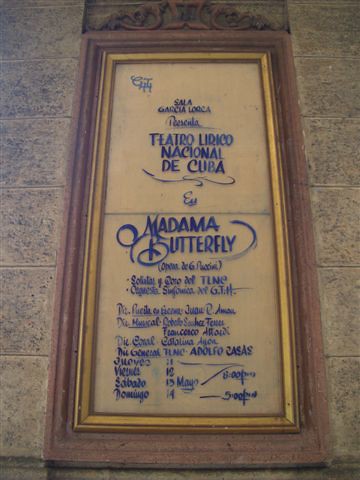The image depicts a detailed sign set against a concrete wall, with visible stone blocks to its left and right. The sign has a long rectangular frame featuring an outer brown border adorned with a delicate design at the top, and an inner gold edging. The sign itself has an off-white or beige background with bold blue lettering. The prominent text at the top reads "Sala Garcia Loca," followed by "Teatro Lirico Nacional de Cuba," suggesting a location or venue. Below, in stylized script, it prominently announces "Madama Butterfly." Additional text below this likely provides further details such as times, dates, or prices, but it is too small to read clearly. Although the sign appears relatively new, the lighting in the area is dim, making certain elements hard to discern.